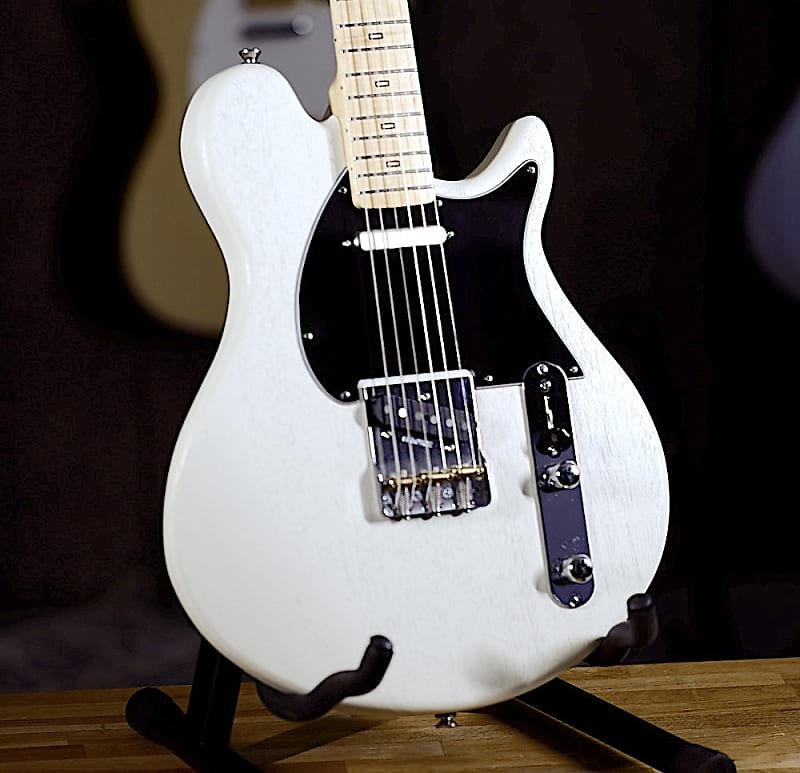A detailed photograph showcases a striking electric guitar with a white body on a sleek black metal stand, placed on a wooden surface. The instrument features a black pickguard, a silver bridge with copper bridge saddles, a black bridge pickup with silver pole pieces, and a narrow white neck pickup resembling a lipstick-style pickup. The neck is made of light maple wood, and the fretboard appears to be of similar material, providing a contrasting visual appeal. Two controls are mounted on a silver plate near the bottom of the guitar, accompanied by a pickup switch.

The background of the image is a black wallpaper with a guitar design, adding an artistic flair to the scene. Behind the primary guitar, there is another guitar visible; it is a brown instrument with a white center, although slightly out of focus. To the right of the main guitar, a yellow guitar with a white pickguard and silver pickup is faintly visible, contributing to the overall depth and context of this visually rich setting.